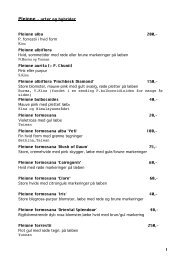The image depicts a very small, low-resolution page, resembling a menu with a white background and black text. At the top, there's a header likely indicating a section such as appetizers, entrees, or desserts. Below the header, the page is organized with several bold subheadings or names of menu items, each followed by a brief description in smaller black text. Descriptions are generally one line long, with a few extending to two lines. On the right-hand side of the page, corresponding to each menu item, are numbers that appear to be prices. Although the fine, blurry print renders the text unreadable, the structured layout suggests it's a list of items, possibly for a restaurant menu, with item names and prices clearly delineated.